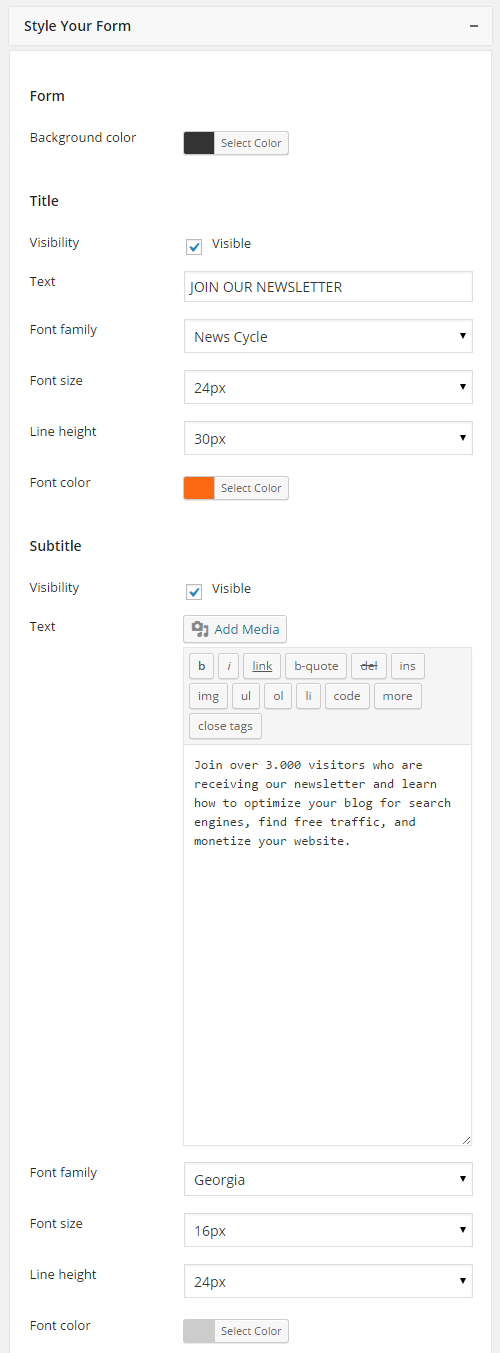Screenshot of a form customization interface titled "Style Your Form." The interface features a white background with a light gray outline on the left, right, and top edges. The form provides various fields for customization, including 'Background Color' (currently set to black). The 'Title' section offers options for 'Visibility,' 'Text,' 'Font Family,' 'Font Size,' 'Line Height,' and 'Font Color,' with the font color set to orange. A 'Subtitle' section follows, presenting similar customization options. There is a visible text box checked, displaying the message: "Join over 3,000 visitors who are receiving our newsletter and learn how to optimize your blog for search engines, find free traffic, and monetize your website."